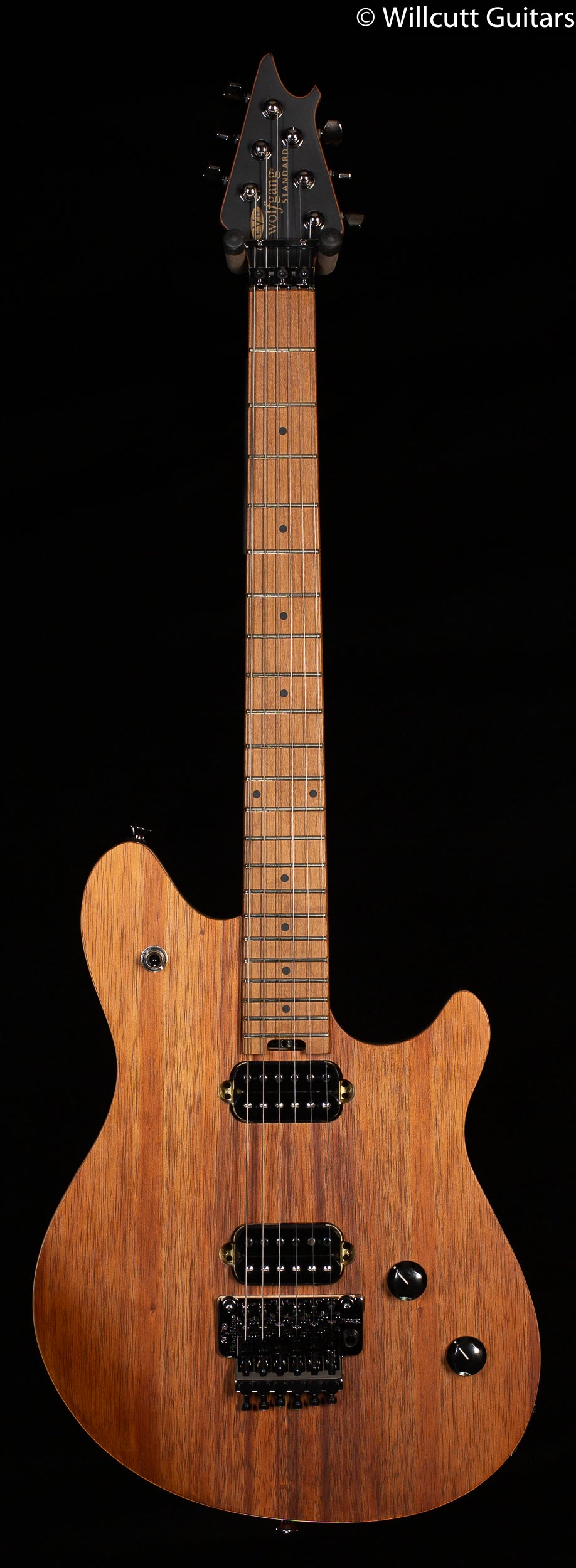This color photo features a beautifully symmetrical electric guitar set against a completely black background. The guitar, crafted from a reddish, creamy, and pale wood that is likely maple, spans the entire horizontal frame of the image. At the top, where the strings are adjusted, the wood transitions to a dark, black section with striking silver details. Throughout the neck of the guitar, small black dots mark the frets. The body of the guitar includes two adjustment knobs and an input jack, indicative of its electric nature. The image composition is clean and focused solely on the guitar, with the only text present in the upper right corner, reading "Will Cut Guitars". This text does not appear on the guitar itself. The overall presentation is professional, showcasing the elegant design and potential high quality of the instrument.